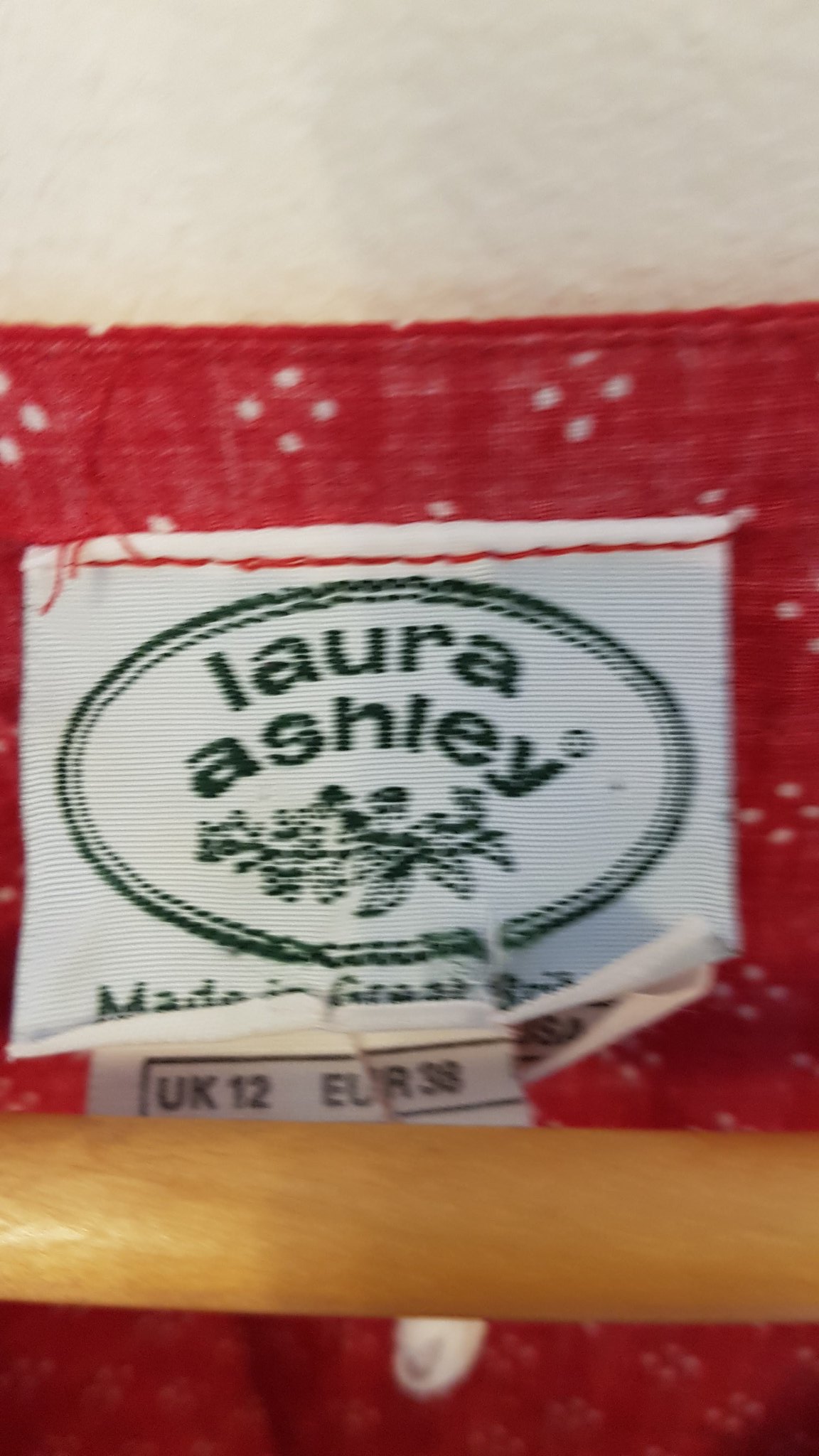This image depicts the back of a red shirt, prominently showcasing its label. The label, in the shape of an oval, features the words "Laura Ashley" along with an illustration of leaves. Below this text, there is additional information, starting with "Made in," but the rest is obscured and unreadable. A side tag is also visible, indicating the sizes "UK 12" and "European 38," although part of this tag is hidden by a wooden pole. The shirt itself is red and adorned with a repeating pattern of four small circles arranged in a diamond shape, creating an intricate and consistent design throughout the fabric.